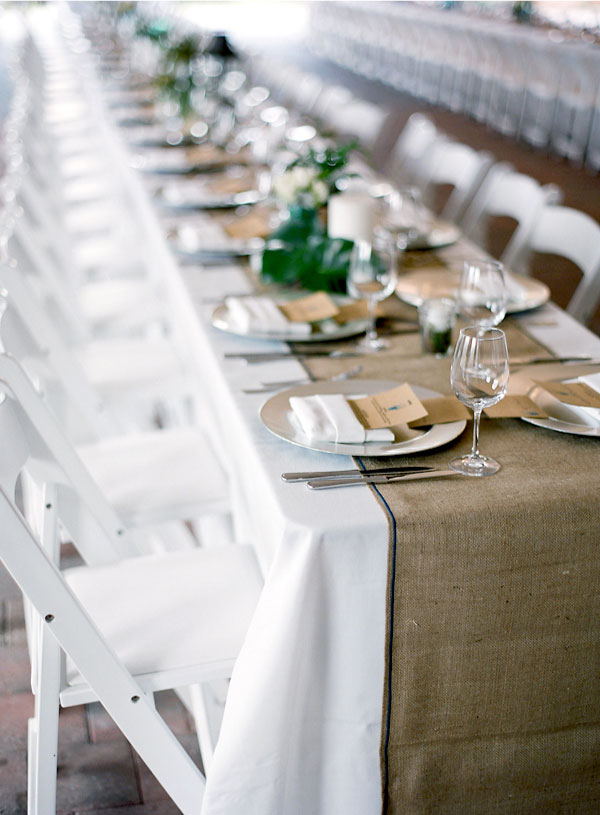This image captures a meticulously arranged setting for a formal event, possibly a wedding or a gala, featuring long rows of tables adorned with white tablecloths. A thinner, brown runner overlays the white tablecloths, adding depth to the elegant display. Each place setting includes a white plate accompanied by neatly folded napkins, each containing a brown slip, likely providing details about the event. Silverware is precisely arranged on either side of the plates, with wine glasses positioned to the upper right. The tables are lined with dozens of white chairs on both sides, and every fourth place setting is punctuated by lush green plants, adding a touch of natural beauty to the sophisticated ambiance. The scene extends into the distance, becoming progressively blurrier, yet maintaining the uniformity of the carefully crafted arrangements. The soft lighting and the hint of additional tables in the background suggest a spacious, inviting atmosphere perfect for a grand celebration.